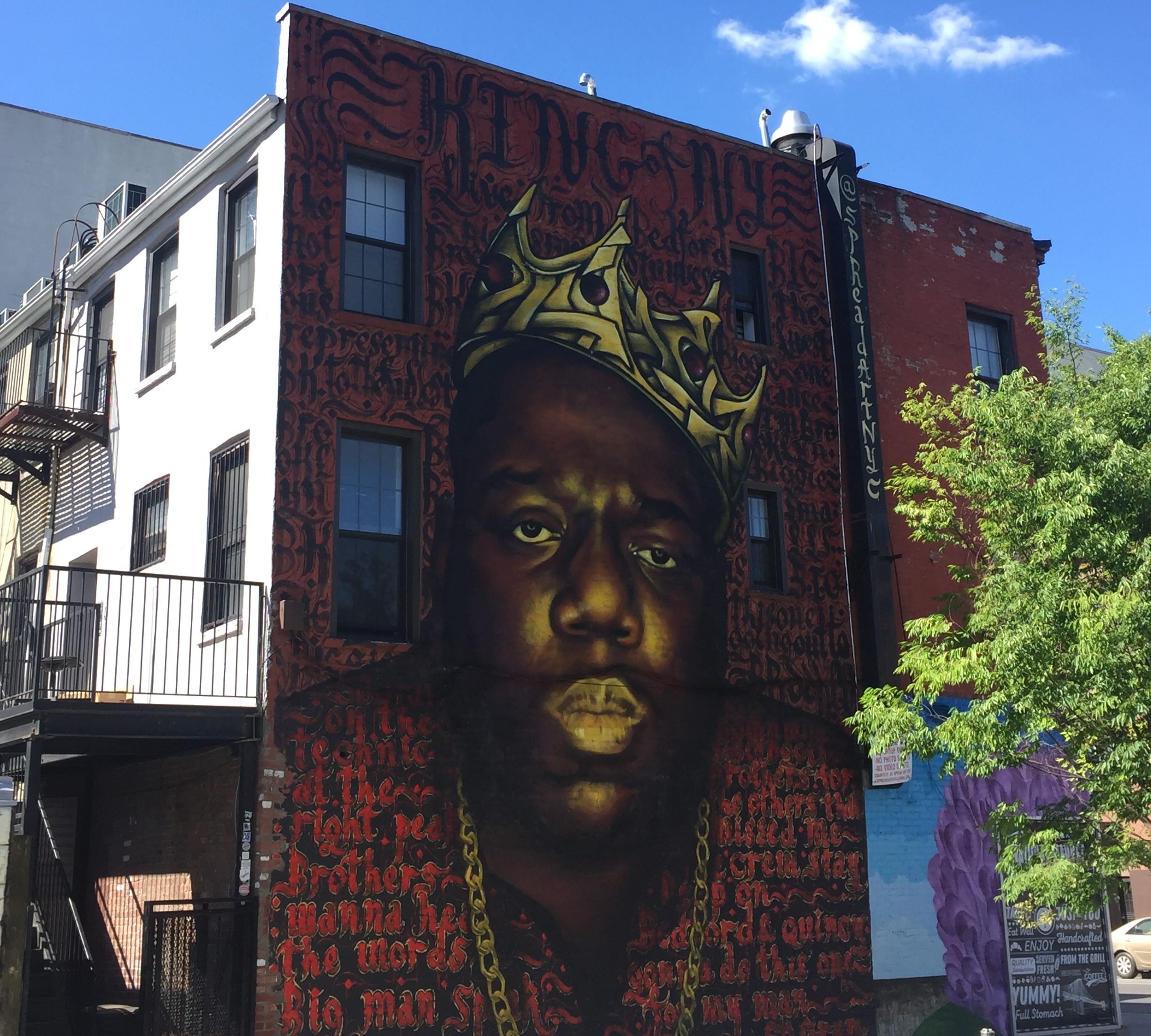The image showcases a vibrant mural on the side of a brick apartment building, possibly located in New York City. The focal point of the mural is an iconic portrait of the rapper Notorious B.I.G. (Biggie Smalls), depicted with a gold crown on his head and a gold chain around his neck. He is dressed in a black top with red text, and his expression appears tired or indifferent. The mural includes intricate graffiti artwork and scattered lyrics, adding layers of detail to the scene. The building itself features multiple rooms, with the mural covering the dark gray and red main wall, while the left side shows a white surface with an external staircase and a deck with metal bars. The words "King of New York, live from Bedford" are prominently displayed on the mural, and a black gutter beside it bears the phrase "spread art New York City." A green leaf tree stands on the far right of the image, set against a blue sky with a single floating white cloud, highlighting the contrast between the urban environment and the natural elements.